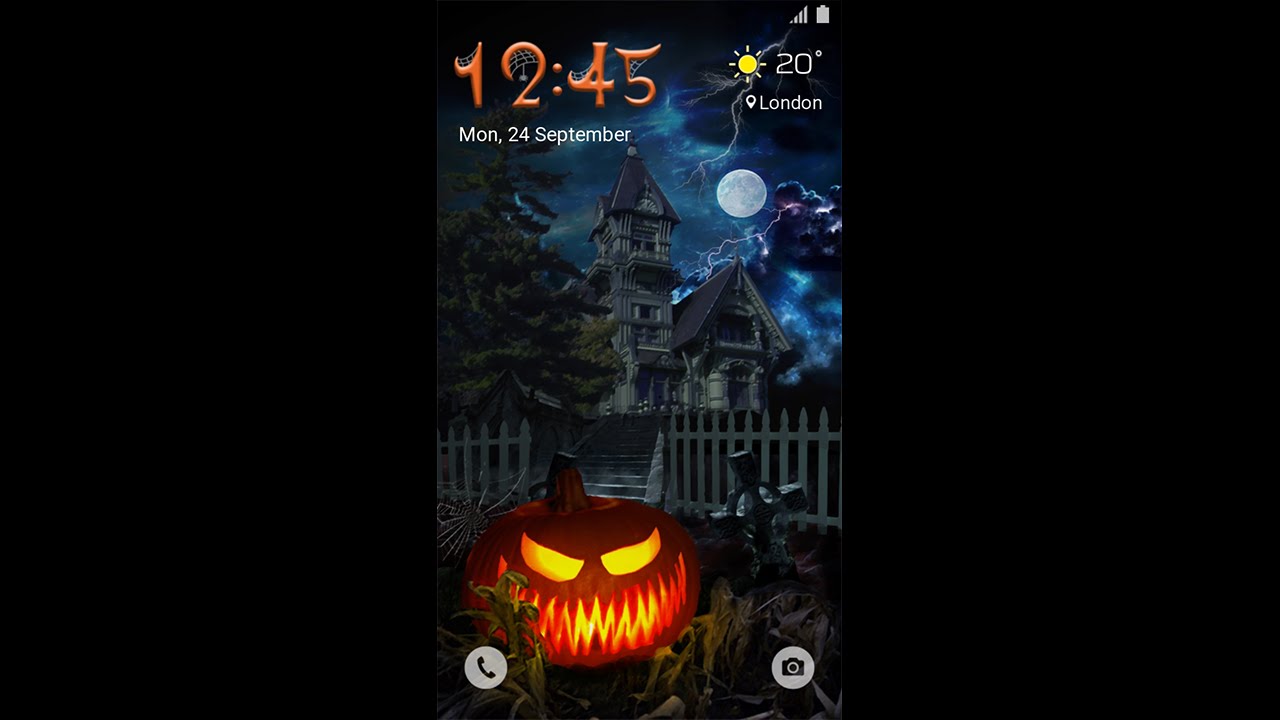This image is a screenshot of a phone screen, displayed in a resized format with large black borders on the left and right sides. The phone's status bar indicates a full battery and a full cellular connection. Below the status bar, there's a sun icon showing a temperature of 20 degrees, accompanied by a location symbol indicating London.

In the upper left-hand corner, the time is displayed as "12:45" in an orange, thin, and spiky font adorned with cobwebs. Directly beneath the time, the date "Monday, 24th September" is written in white font.

The phone's background features a spooky scene of a mansion under a nighttime sky filled with clouds, lightning, and a full moon. A dark green tree stands to the side of the mansion, which appears to be three or four stories tall, with a pointed spire and a slanted roof. A grey staircase leads up to the mansion, which is enclosed by a grey picket fence.

At the bottom of the screen, a glowing orange jack-o-lantern with sharp, spiky teeth and pointy eyes adds to the eerie atmosphere. To the right of the jack-o-lantern, there's a cross-shaped tombstone, completing the spooky Halloween-themed aesthetic.